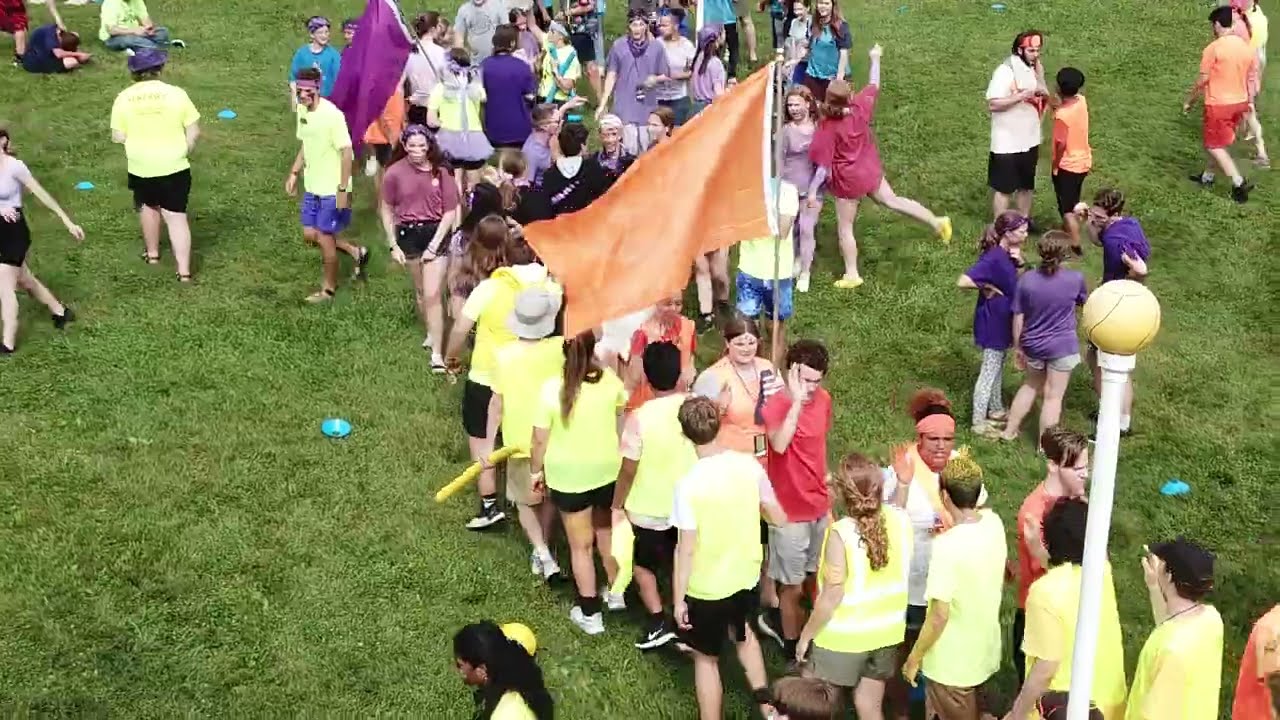The image is an aerial shot taken from a low height, capturing a green grassy field populated with multiple groups of people. In the foreground, starting from the lower right-hand corner and stretching diagonally towards the center, there's a single file line of kids dressed in bright yellow shirts and vests. The first person in this line is holding a yellow baton-like object. Adjacent to this group, on the right-hand side, stands a tall white pole about twice the height of the kids, topped with a ball.

The yellow-clad kids appear to be part of a coordinated activity, possibly a team event. They are contrasted by another group of people walking in the opposite direction, seemingly composed of individuals in regular street attire, suggesting they might be observers or participants from a different activity. Some members of these groups are seen engaging in high-fives, conveying a sense of camaraderie or post-game congratulations.

Scattered throughout the field, there are other individuals wearing purple and orange shirts, creating a colorful scene. Teal discs are randomly placed on the field, hinting at a game or activity setup. In the center of the photo, a prominent orange flag is visible, while towards the left, a purple flag can be seen, adding to the vibrant atmosphere of the scene.